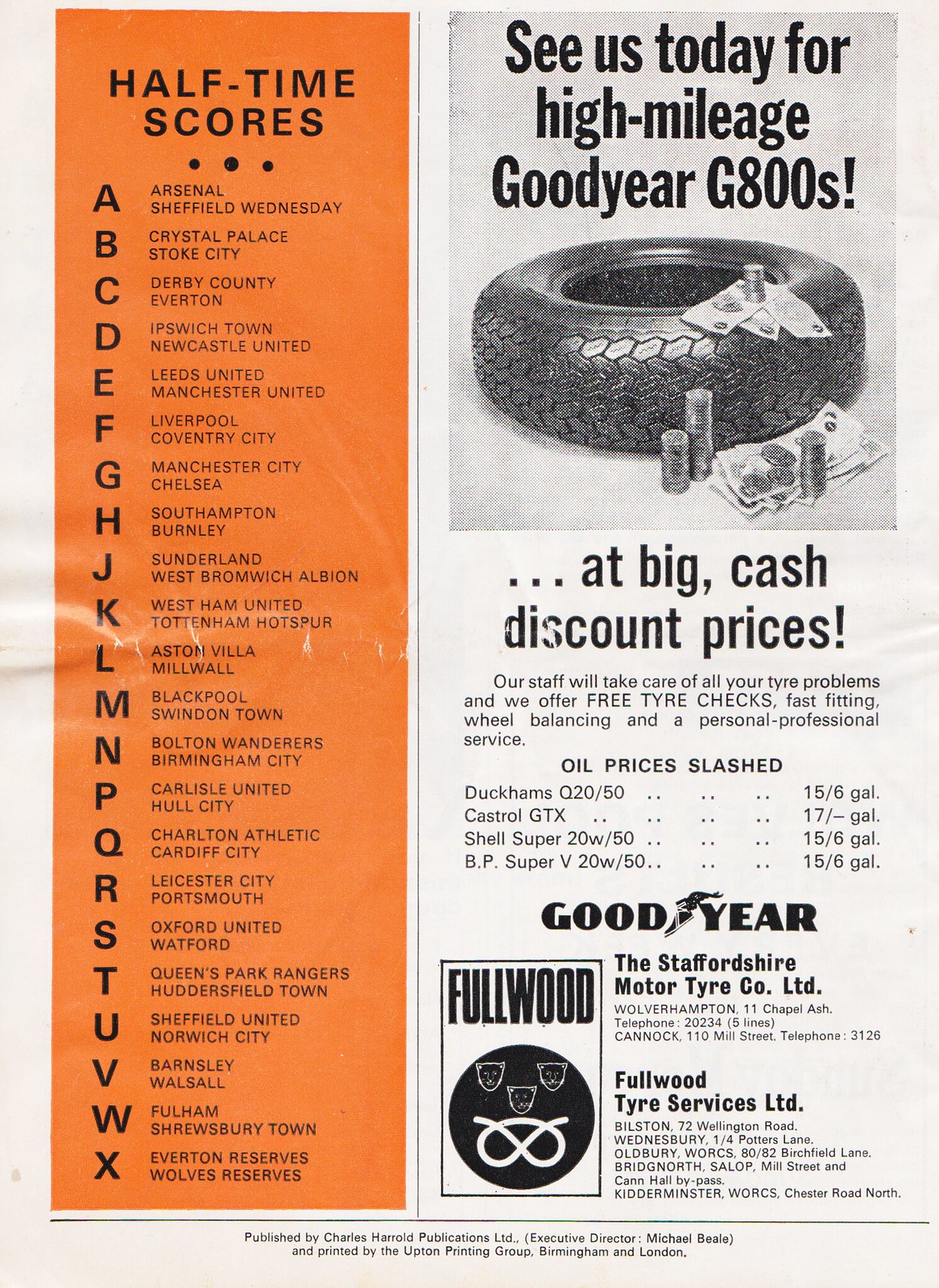The image showcases a vintage advertisement, divided into two distinct panels. The left panel, predominantly orange, features a printed schedule of halftime scores for various English football matches organized alphabetically. For example, Arsenal versus Sheffield Wednesday, Crystal Palace versus Stoke City, and others, each denoted by letters A through X. The right panel, set against a white background, displays an advertisement for Goodyear tires. The ad highlights a high mileage Goodyear G800 tire available at big cash discount prices, accompanied by a detailed list of oil prices that have been slashed, including brands like Duckhams and BP Super. The ad also emphasizes the company's professional service offerings such as free tire checks, fast fitting, and wheel balancing. The advertisement is from the Staffordshire Motor Tire Company Limited, based in Wolverhampton with additional locations including Cannock. Contact details for these locations are also provided in the ad.